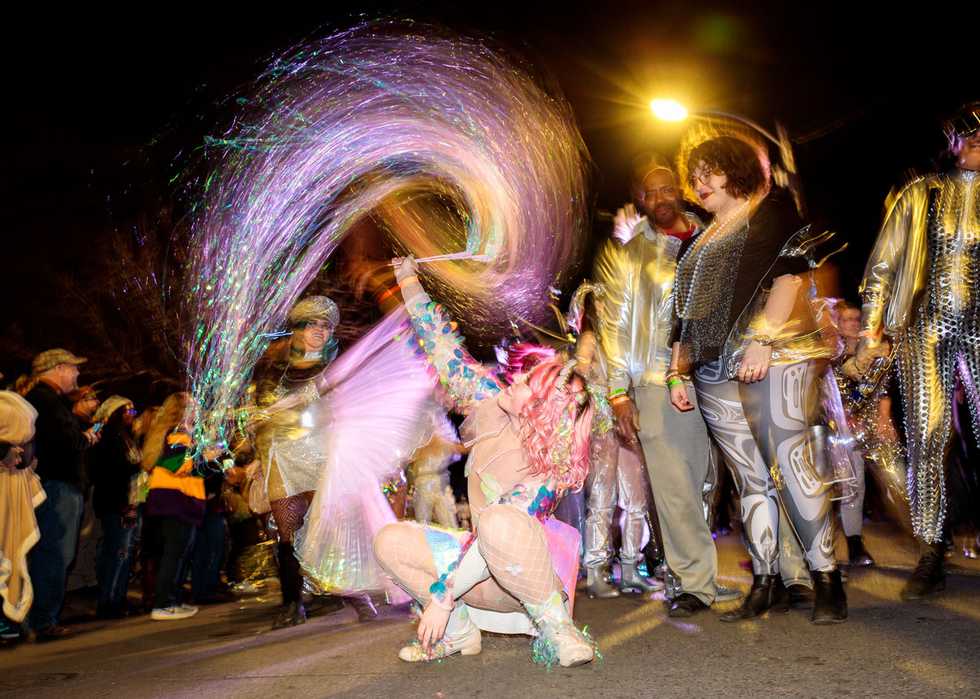This image, taken at nighttime, captures the vibrant energy of a parade. The photograph, shot from a low angle, reveals a parade scene unfolding on a street, filled with spectators lining the sides. Dominating the center is a woman crouching on the street, dressed in a rainbow-colored outfit adorned with green fishnets and a pink skirt. She has striking pink hair, possibly a wig, and waves a stick affixed with long, hair-like colorful strands resembling a horse's mane, capturing the sparkling motion mid-swing. To her left stands an African American man and a white woman dressed in a black top and silver pants, while on the far right, a man clad in a solid metallic bodysuit that resembles snake scales adds to the festive spectacle. The dark background contrasts sharply with the colorful costumes, making the parade's lively spirit pop against the night sky.